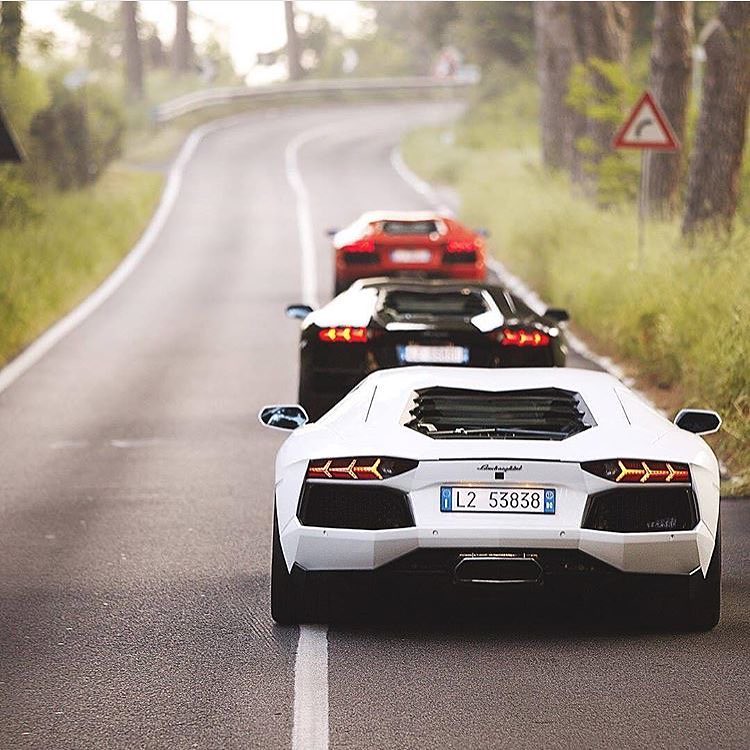The image depicts a scenic outdoor roadway flanked by tall, lighter green grass and tree trunks, evoking a woodsy, almost forest-like atmosphere. It's bathed in a soft golden light, suggesting it might be taken during the golden hour, with sun rays filtering through the trees in the blurred background. On the right side of the road, lined up in single file and traveling away from the viewer, are three distinct sports cars, believed to be Lamborghinis. The foremost car is red, followed by a black one, and the last is white. The license plate of the white car reads L253838. All vehicles seem to be braking, as indicated by their illuminated brake lights. To the right side of the road, embedded in the grassy area, there's a road sign featuring a red triangle with a white background and a black curved arrow, indicating a turn ahead.